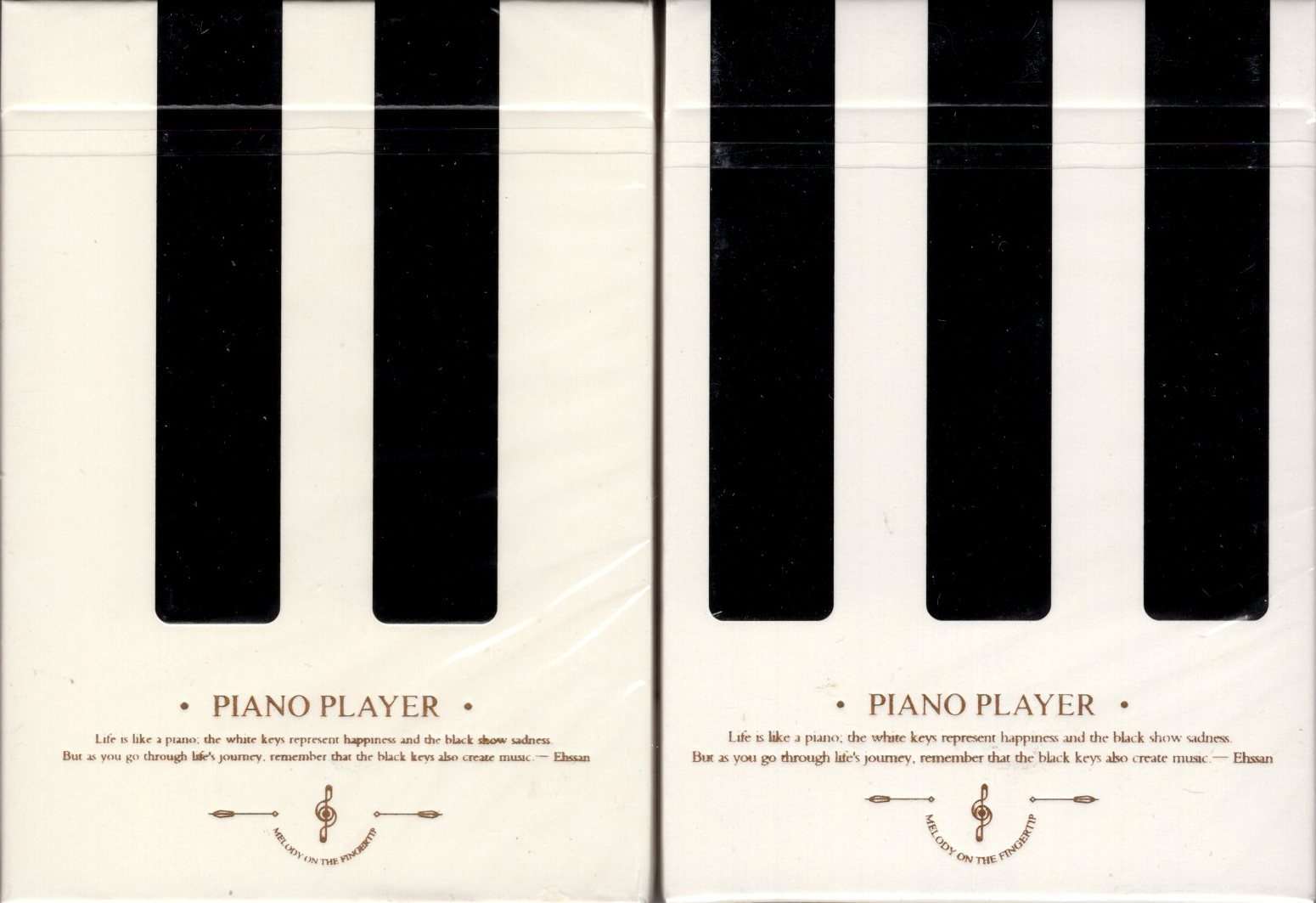The image is divided down the middle into two sections that resemble pages of an open book, with a predominantly white background featuring simple graphics of piano keys. The left section contains two black piano keys descending from the top, while the right section displays three black piano keys. 

Both sections are labeled with the phrase "Piano Player" in dark lettering at the bottom. Below this, an identical inspirational quote is printed on each side: "Life is like a piano. The white keys represent happiness, and the black show sadness. But as you go through life's journey, remember that the black keys also create music."

There is additional text below the quote in a curved format that states, "melody on the fingertip," accompanied by an illustration of a musical note with lines that resemble arrows pointing in different directions. The image appears to be a scan of a wrinkled piece of paper, with subtle indications that it might be mounted or painted on a wall.